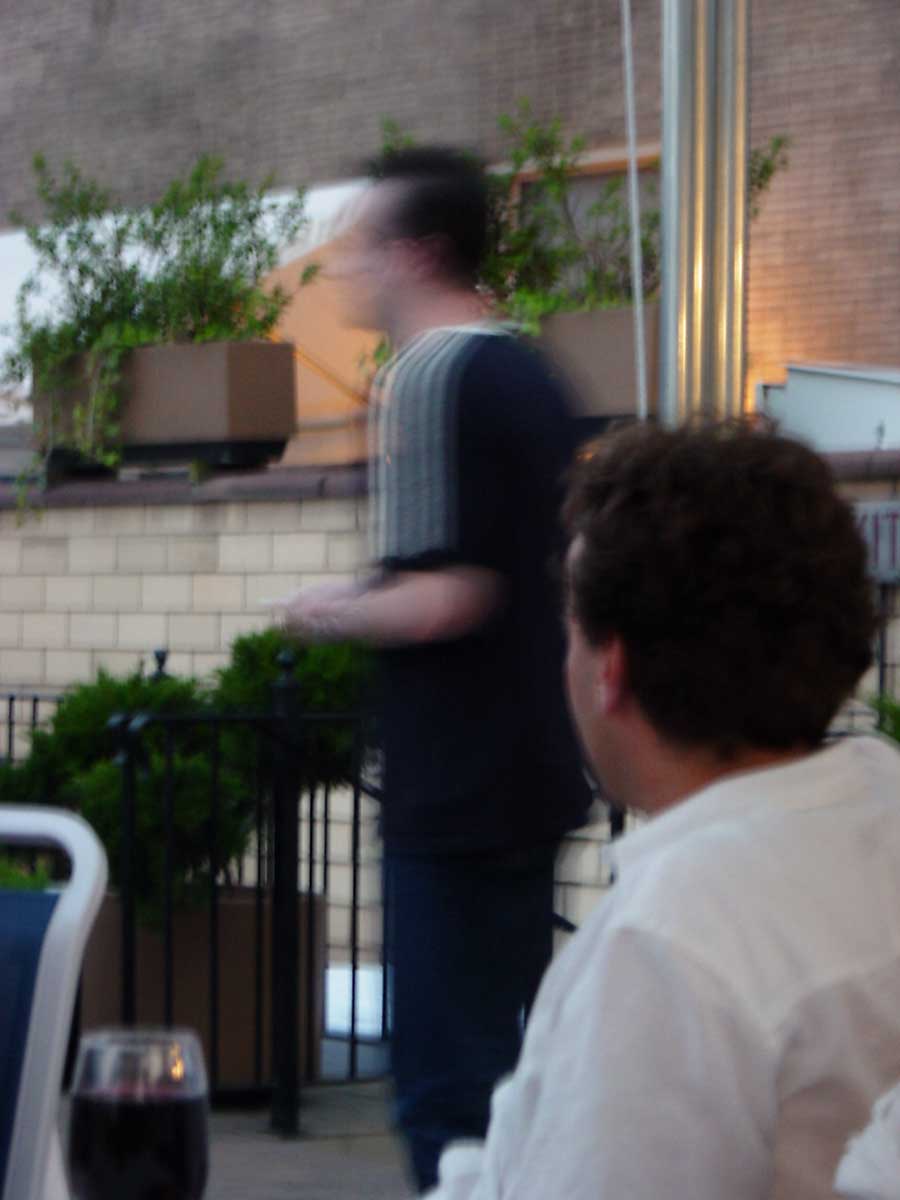In this image, two men appear to be engaged in a conversation, presumably in an outdoor venue. The primary focus is on a Caucasian male with black hair, wearing a dark blue or black shirt adorned with white stripes along the sleeves and possibly a white collar. Although he is slightly out of focus, his attentive posture suggests he is listening intently. Seated nearby, another man dressed in a white shirt is looking in the direction of the first, though his face is not clearly visible. The setting seems to be a backyard or a hotel balcony, characterized by a brick wall and surrounded by various planters and potted plants. A glass of wine sits on the table, adding a casual, relaxed atmosphere to the scene.